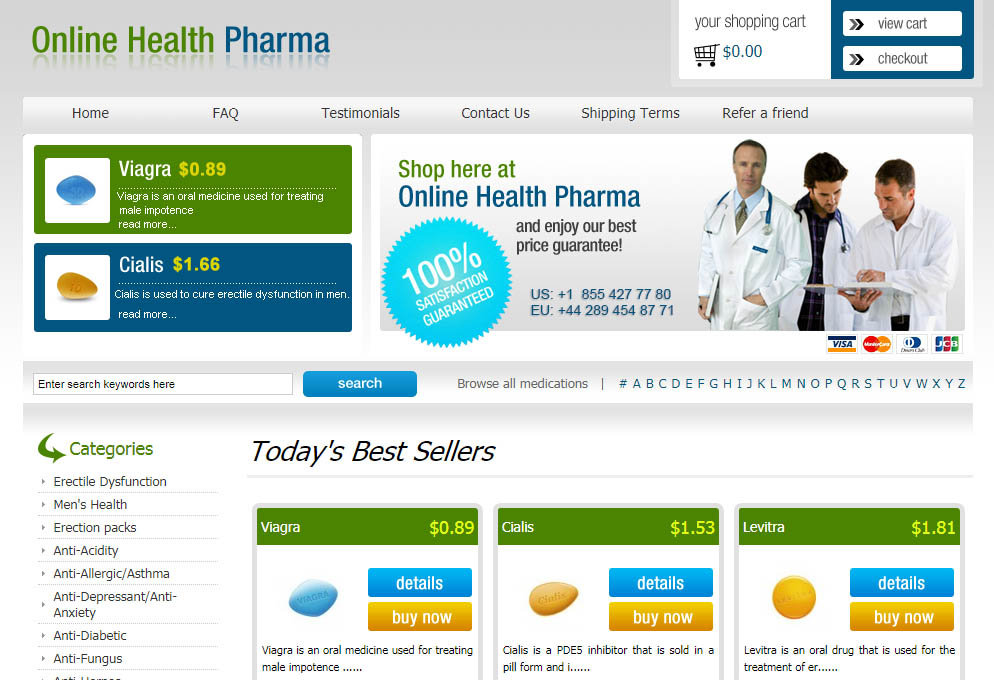The website banner features a large, gray area at the top. Starting with green text, the words “Online Health” appear prominently, with “O” and “H” capitalized. Beside it, the word "Pharma" is displayed in blue, complete with a subtle reflection, though not all letters reflect uniformly. 

On the right side of this gray area, there's a white square containing black text and an icon of a shopping cart. The text indicates "Your Shopping Cart" with a displayed amount of "$0.00," signifying an empty cart. Within this same section, a small dark blue rectangle houses two buttons, each beginning with an arrow, one gray and one black. The first button reads "View Cart," while the second says "Checkout."

Floating within the gray banner, a mid-gray rectangle presents several navigation options in black text: Home, FAQ, Testimonials, Contact Us, Shipping Terms, and Refer a Friend.

To the left, against a lighter gray backdrop, there’s a dark green rectangle showcasing a blue Viagra pill. Beside it, white text spells out "Viagra," with the price "$0.89" in yellow. Below this, white text describes Viagra as "an oral medicine used for treating male impotence," followed by "Read more…" in an ellipsis.

Further down, a blue rectangle features an orange, teardrop-shaped Cialis pill marked with the number "10." Next to the pill, "Cialis" is written in white, with the price "$1.66" in yellow. A brief description states, "Cialis is used to cure erectile dysfunction in men," followed by "Read more…"

Adjacent to these product descriptions, two doctors are shown examining a chart and engaging in conversation, both donned in white lab coats. One doctor sports a plaid shirt, while the other wears a white dress shirt with black dress pants. Facing the camera is another doctor in a cyan blue dress shirt with a dark tan tie, also wearing a white lab coat and stethoscope. He holds a book and has short black hair, appearing to be middle-aged.

In the lower left corner, a green text label with an arrow points to a rectangle titled "Categories." The following categories are listed in black text with gray arrows: Erectile Dysfunction, Men's Health, Erection Panics, Anti-Acidity, Anti-Allergy/Asthma, Anti-Depressant/Anti-Anxiety, Anti-Diuretic, and Anti-Fungal. An additional "Anti-" category is slightly cut off at the bottom.